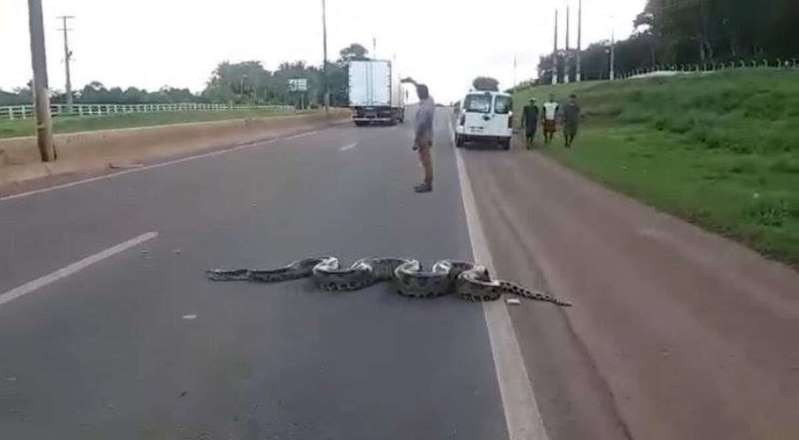This detailed photograph captures a potentially six or seven-foot-long python, characterized by its grayish color with black splotches, as it slithers across a two-lane road. The snake is primarily in the right-hand lane but its tail extends onto the shoulder. Packed into an S shape, the python's head is facing towards the center line of the road. In the background, a man appears to be taking a selfie with the snake, and three others are visible walking along the grassy side of the roadway towards the python. The right side of the image features a white van and a cluster of grass and trees, along with a few telephone poles. Further up the road, a large white moving truck can be seen parked on the road, adding to the scene's dynamic backdrop. The composition emphasizes the snake's impressive presence and the human activity surrounding it.